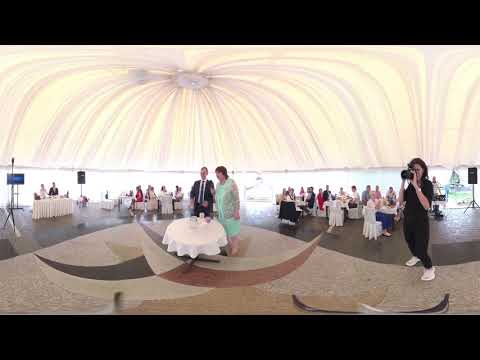This detailed photograph captures a vibrant celebration, likely a wedding, set inside a large hall with a curved, dome-like, cream-colored ceiling. The image, taken with a fisheye lens or similar effect, exhibits slight curvature and black horizontal strips at the top and bottom, adding to its unique perspective.

In the center of the image stands a small, circular table draped in a white cloth, around which a man and woman are positioned. The man, clad in a black suit, white shirt, and black tie, stands on the left, while the woman on the right wears a striking green dress. An item rests on the table, though it remains indistinct due to blurriness.

Adjacent to the central couple, a female photographer dressed in a black shirt, black pants, and white shoes is intently capturing the scene. Surrounding tables and chairs, some ornate or finely detailed, are occupied by guests, contributing to the lively atmosphere. The floor beneath features an intricate design in black, red, and cream hues, harmonizing with the hall's elegant aesthetic.